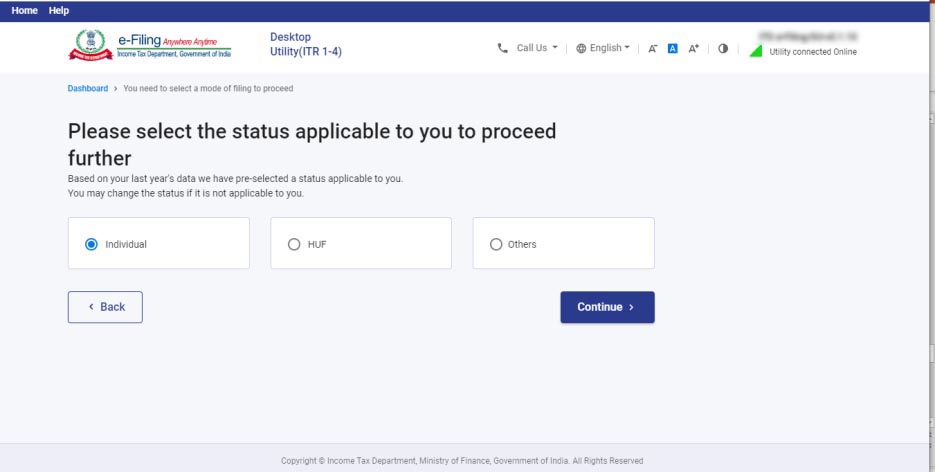The image appears to be a screenshot from an online tax filing service, specifically from the Income Tax Department of the Government of India, likely provided by the IRS or a similar tax authority. 

At the top of the interface, there is a solid blue navigation bar featuring two options on the left: "Home" and "Help." Below the navigation bar is the company logo, which includes a green circle with a red banner underneath containing some indistinguishable elements. The company's name, "e-filing," is displayed in blue text accompanied by the slogan "Anywhere, Anytime" in red text. Directly beneath this is a solid green line separating the header from the main content, with the words "Income Tax Department, Government of India" written beneath it.

Adjacent to the logo are additional options, including "Desktop" and "Utility." As you move to the right, there is a "Call Us" button with a phone icon, a language selection feature set to English, a font adjustment option, and a final option labeled "Utility Connected Online."

Underneath this header, the main content begins with the heading "Dashboard" in blue text. Below this heading, the interface prompts the user to "Select a mode of filing to proceed." In bold letters, it instructs the user: "Please select the status applicable to you to proceed further," followed by a smaller note indicating: "Based on last year's data, we have pre-selected a status applicable to you. You may change that status if not applicable to you." 

Currently, the selected status is "Individual," indicated by a filled blue circle. The other available status options, "HUF" (Hindu Undivided Family) and "Others," are not selected.

At the bottom of the screen, there are navigation buttons: to the left is a white "Back" button, and to the right is a solid blue "Continue" button.